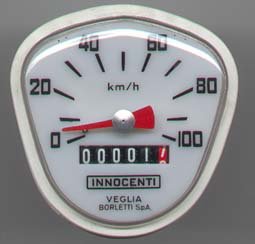A square photo captures a detached motorcycle speedometer against a gray background. The speedometer, encased in white plastic, features a clean white face with calibrated displays. It measures speeds from 0 to 100 kilometers per hour, with marked intervals at 0, 20, 40, 60, 80, and 100 km/h, and smaller lines denoting intermediary speeds. Positioned centrally below the numbers is the "KM/H" notation. The speedometer's needle, which is red with a silver center, prominently stands against the white backdrop. Additionally, a tachometer is visible, showing a reading just past 1.7 kilometers. The brand "Innocenti" is clearly inscribed on the face, hinting at Italian origins, and beneath it, the name "Veglia Borletti"—likely the manufacturer of the instrument.